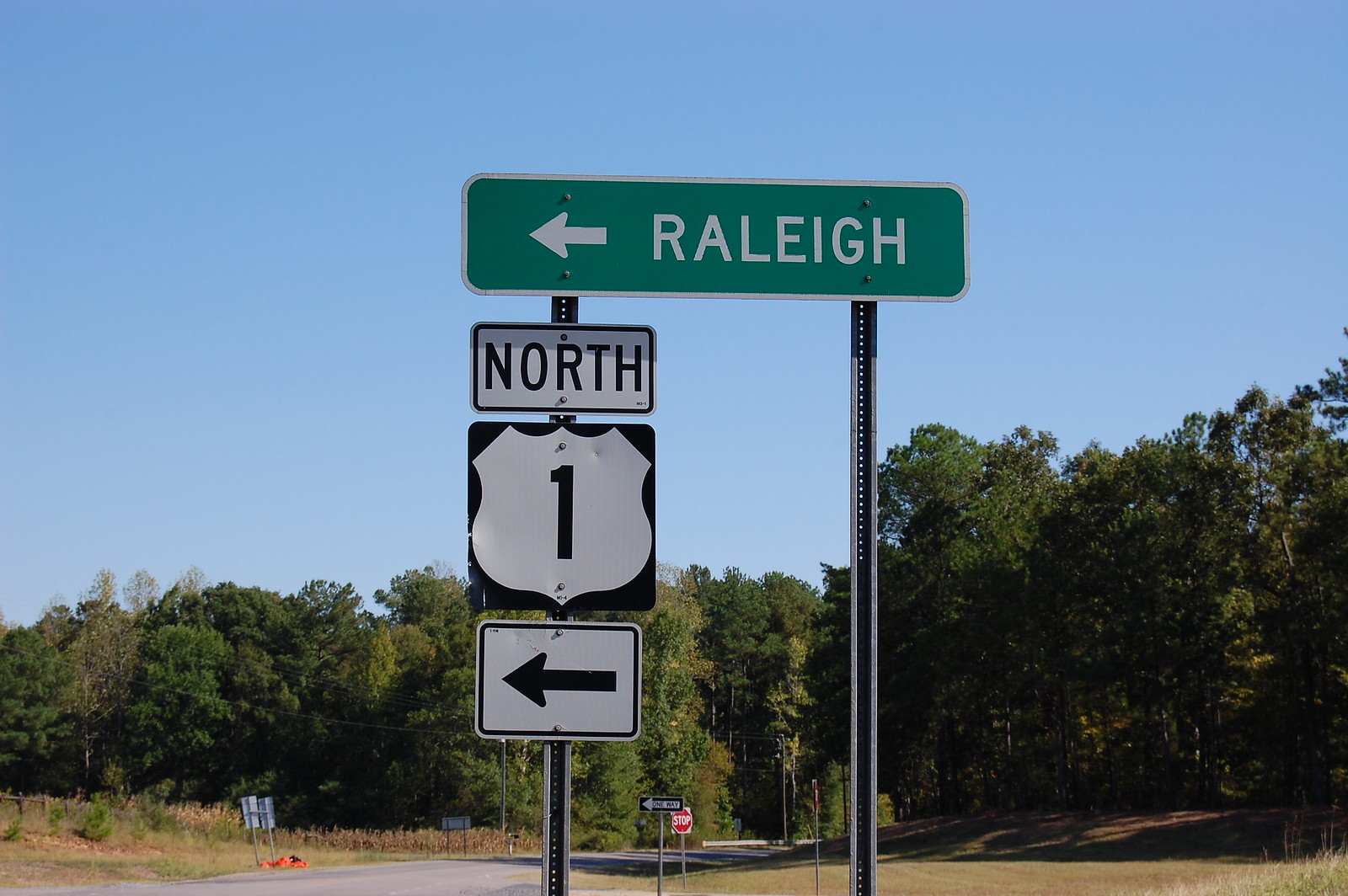The image depicts a green street sign indicating "Raleigh" with an arrow pointing to the left, signifying the direction towards Raleigh, North Carolina. Below this, there's a U.S. Highway sign with the number "1" and the word "North" above it, also pointing to the left. The highway sign features black lettering on a white background. Below these signs, the lower portion of the image shows a stretch of road. On the left side of the road lies an orange jacket or similar item next to a smaller, unidentifiable sign. Centrally, there is a visible stop sign accompanied by a one-way sign directing traffic to the left. Occupying approximately half of the image from top to bottom is a dense cluster of dark green trees in full bloom. The upper portion of the image showcases a clear, cloudless blue sky, emphasizing the bright and pristine weather conditions.